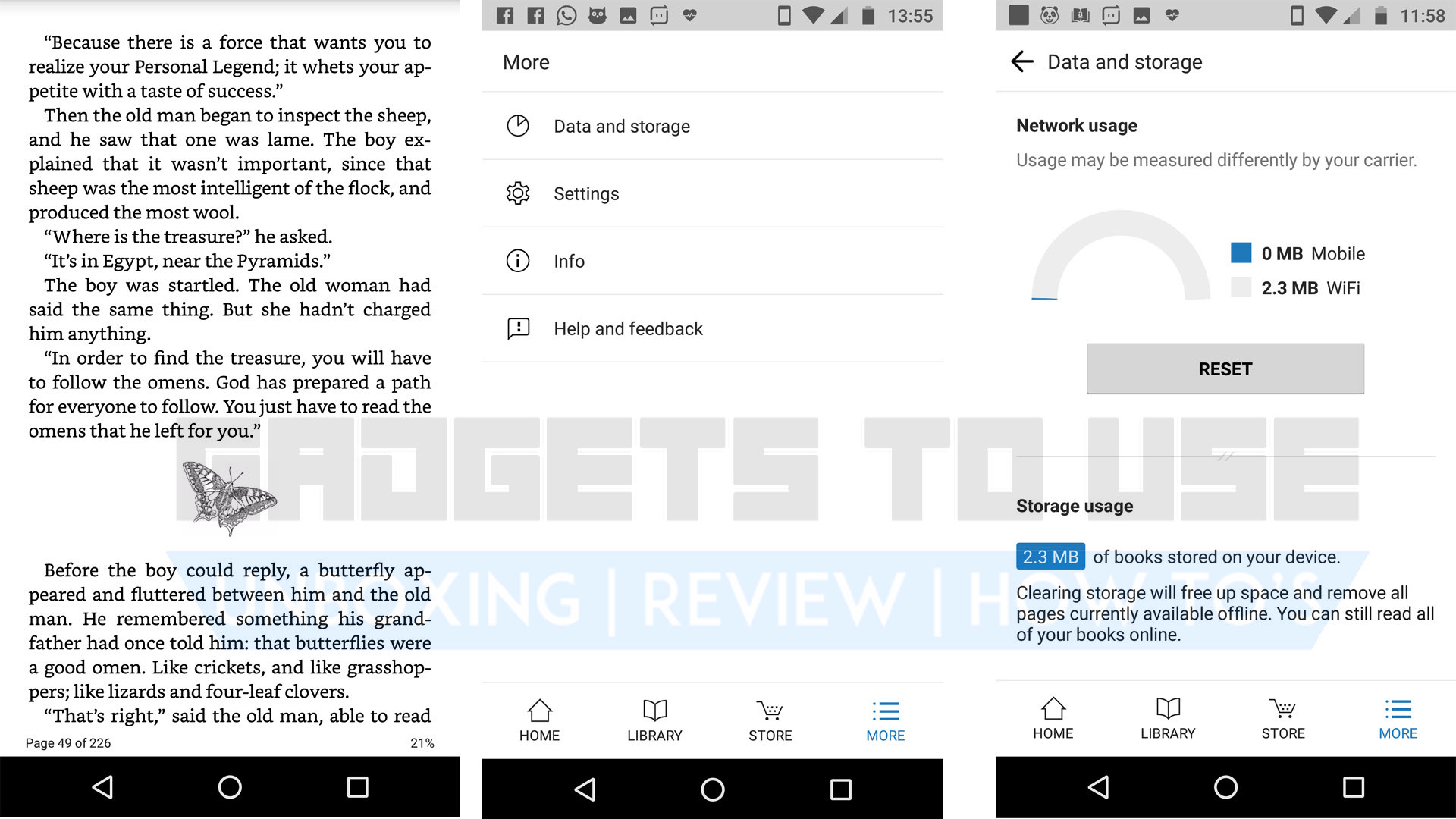The image showcases three distinct screenshots from a mobile device, each set against a white background with a watermark reading "Gadgets to Use Review" partially obscured by text. The leftmost screenshot appears to be an excerpt from an article, with readable text filling the screen. The center screenshot displays a settings menu from an application. At the top of this menu is the word "More," followed by several options: a clock or pie chart icon labeled "Data and Storage," a gear icon labeled "Settings," an eye icon labeled "Info," and a chat bubble icon labeled "Help and Feedback." The rightmost screenshot focuses on "Data and Storage" settings, showing "Network Usage" accompanied by a visual chart or meter, along with an option to reset the data usage statistics.